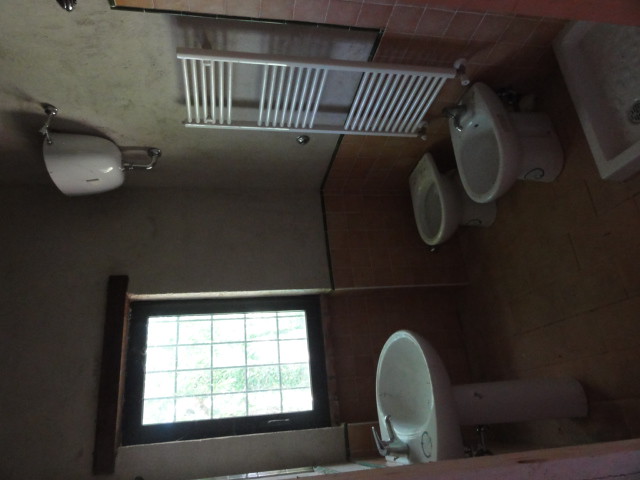This is a sideways horizontal photograph of an old, somewhat dingy bathroom with minimal lighting, suggesting it might be early morning or late afternoon. The primary light source is a window with a grid design of four rows and five columns. The white ceramic sink, featuring a silver metal faucet, is situated along the bottom edge of the sideways picture, with its pedestal on the right. Opposite the sink, located on the left side of the rotated photo, are a pair of fixtures: a squat toilet and a bidet, positioned closely together. Above these fixtures, a white rack, possibly for towels, casts a shadow against the cream-colored wall, indicative of the minimal light streaming in from the window. This wall holds a thin black tile border separating the white upper half from the coral-pink tiles below. The bathroom floor is also tiled in a lighter color, though it's not clearly visible due to the image’s darkness. Additionally, at the angular bottom right, a glimpse of a shower floor reveals a small white-tiled area. The overall atmosphere of the bathroom is dampened further by the poorly lit and potentially outdated conditions, compounded by the unusual angle at which the photograph is taken.